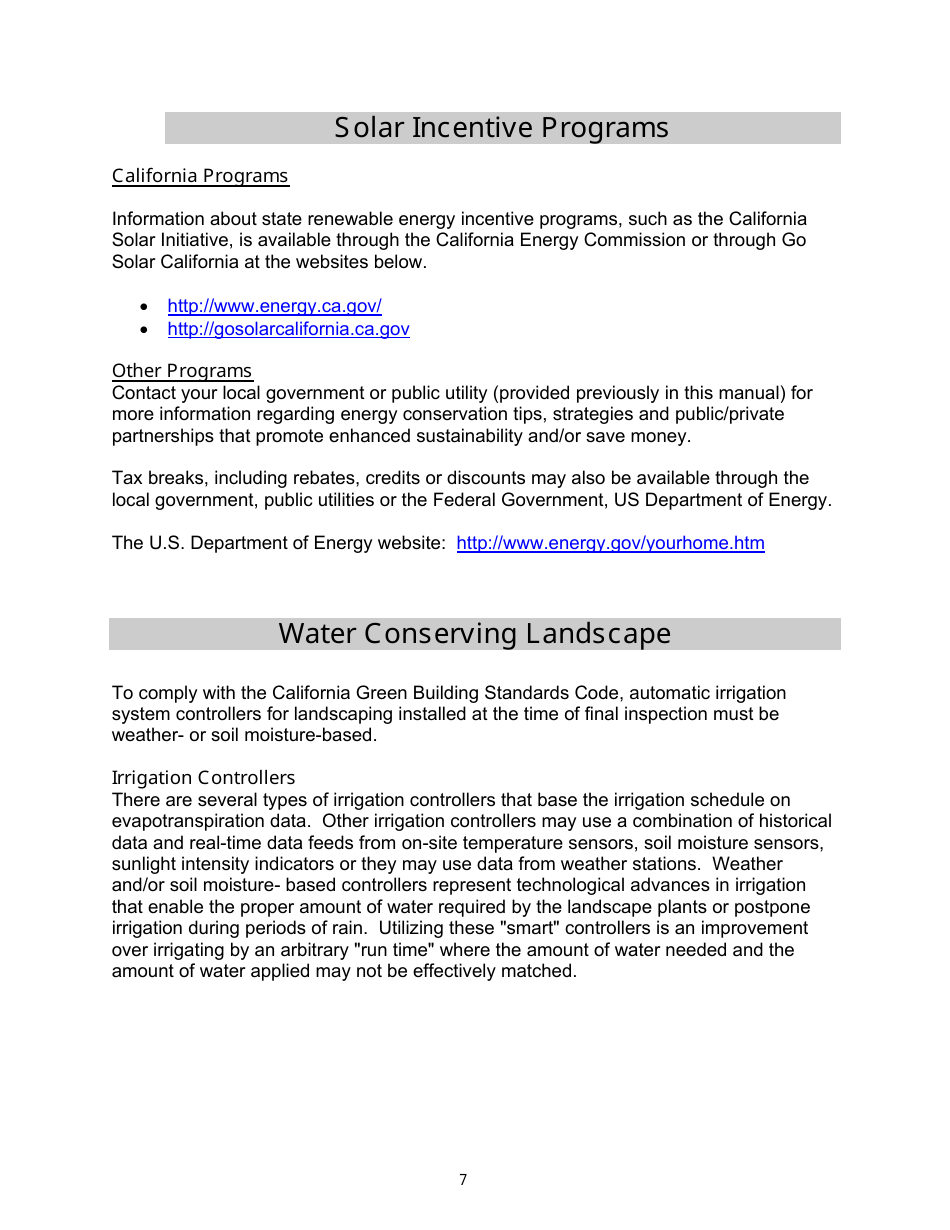**Caption:**

This image highlights a screenshot containing purely informational content about solar incentive programs and water-conserving landscape measures.

**Solar Incentive Programs:**
- **Header:** "Solar Incentive Programs" in a gray rectangle.
- **Section Title:** "California Programs" (underlined).
  - **Text:** "Information about state renewable and energy incentive programs, such as the California Solar Initiative, is available through the California Energy Commission or Go Solar California at the websites below:"
    - [energy.ca.gov](energy.ca.gov)
    - [gosolarcalifornia.ca.gov](gosolarcalifornia.ca.gov)

- **Section Title:** "Other Programs" (underlined).
  - **Text:** "Contact your local government or public utility (provided previously in this manual) for more information regarding energy conservation tips, strategies, and public-private partnerships that promote enhanced sustainability or save money. 
    - **New Paragraph:** "Tax breaks, including rebates, credits, or discounts, may also be available through local government, public utilities, or the federal government (U.S. Department of Energy). Visit [energy.gov/yourhome.htm](energy.gov/yourhome.htm) for more information."

**Water-Conserving Landscape:**
- **Header:** "Water-Conserving Landscape" in a gray rectangle.
  - **Text:** "To comply with the California Green Building Standard Code, automatic irrigation system controllers for landscaping installed at the time of final inspection must be weather- or soil moisture-based. These irrigation controllers use evapotranspiration data, a combination of historical data and real-time data from on-site temperature sensors, soil moisture sensors, sunlight intensity indicators, or weather stations."
  - **Additional Paragraph:** "Weather- and soil moisture-based controllers represent technological advances in irrigation that supply the proper amount of water required by landscape plants or postpone irrigation during periods of rain. Utilizing these smart controllers improves upon arbitrary run-time irrigation, where the water needed and the water applied may not effectively match."